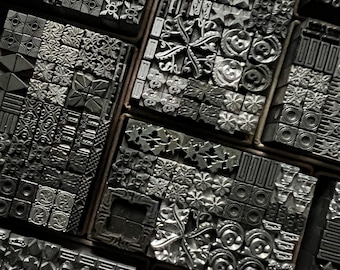This black and white overhead photo showcases an array of tiny metal stamps designed for printing or letter stamping. Arranged in individual boxes, these stamps are meticulously lined up in rows both horizontally and vertically for organized storage. Each stamp features one of various intricate designs—stars, florets, circles, X's, and filigree patterns—crafted from metal in different shades of silver and gray. Some stamps display numeric characters or simple shapes like dashes and asterisks, while most exhibit elaborate decorative or pictorial designs. Notably, every four adjacent stamps seem to form a specific image or pattern, enhancing their visual appeal. Despite their small, square size, these stamps serve a versatile purpose, catering to the artistic preferences of those using them for hand stamping, printing, or decorative projects.